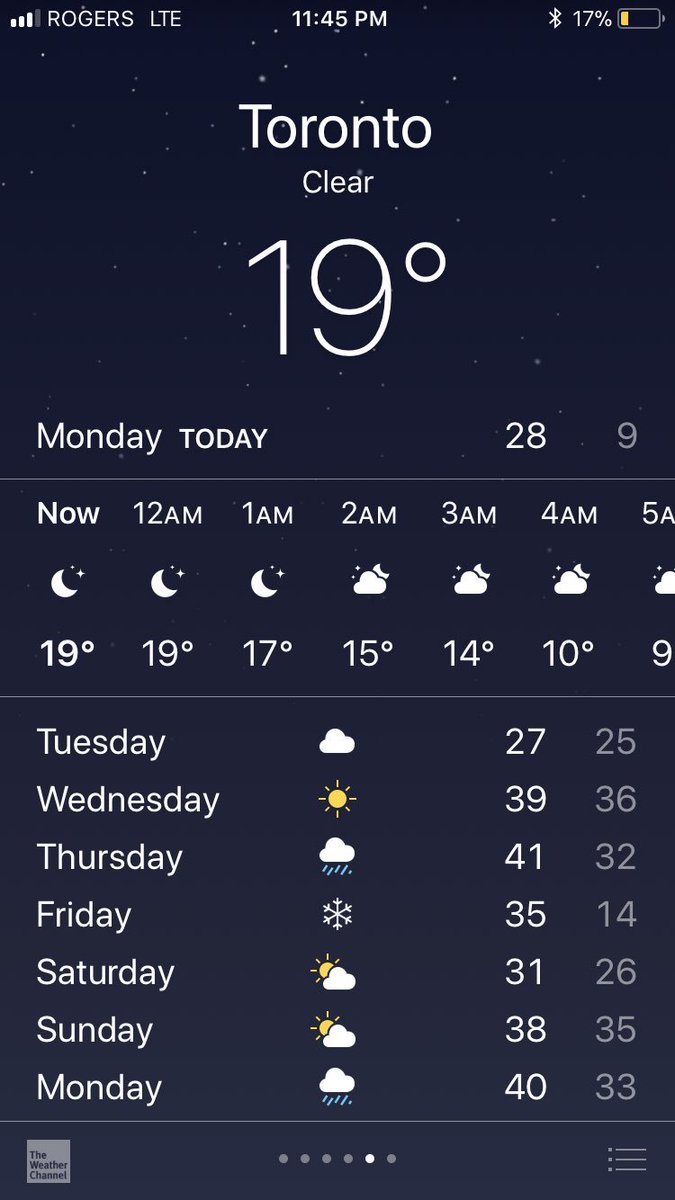Caption: 

The image shows the home screen of a Rogers LTE smartphone at 11:45 PM, connected via Bluetooth with a battery remaining at 17%. The weather forecast for Toronto is currently clear with a temperature of 19 degrees (unit unspecified). It's Monday night, and the forecast details for the coming days are displayed. The hourly forecast shows conditions from midnight through to 5 AM:

- Midnight: Clear
- 1 AM: Clear
- 2 AM: Clear
- 3 AM: Clear
- 4 AM: Clear
- 5 AM: Clear

For the week ahead:

- Tuesday: Cloudy
- Wednesday: Sunny
- Thursday: Mostly cloudy with rain
- Friday: Snow
- Saturday: Partly sunny with lots of clouds
- Sunday: Similar to Saturday with a mix of sun and clouds
- Monday: Like Wednesday, mostly cloudy with definite rain predicted

This thorough depiction conveys both the immediate and upcoming weather conditions.